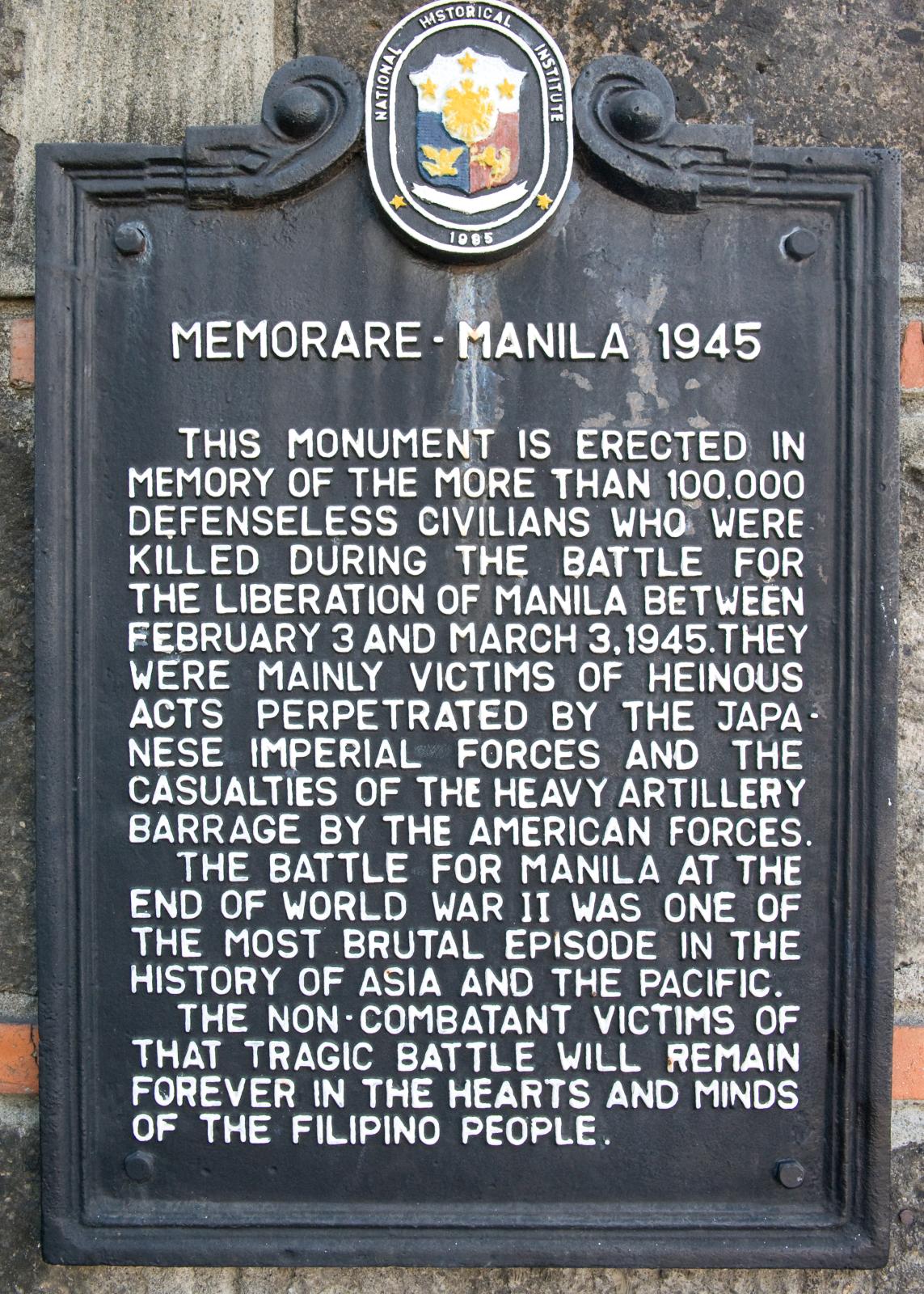The image shows a commemorative plaque set against a backdrop of a brick wall. The black, square plaque features an ornamental design at the top and a central insignia, under which is written in white lettering: "Memorare Manila 1945." Above the inscription, a coat of arms is prominently displayed, labeled with the National Historical Institute. The plaque's text solemnly honors the more than 100,000 defenseless civilians who perished during the Battle for the Liberation of Manila between February 3 and March 3, 1945. These victims suffered due to heinous acts by the Japanese Imperial Forces and the heavy artillery barrage from American forces. The inscribed memorial notes that this event, one of the most brutal and tragic episodes in the history of Asia and the Pacific during World War II, indelibly marks the collective memory of the Filipino people, who hold these noncombatant victims forever in their hearts and minds.